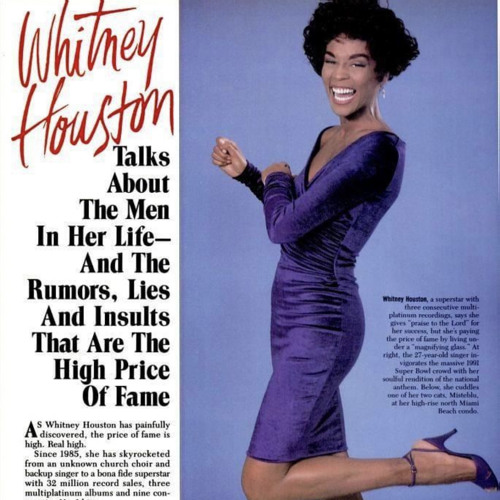This image is a nostalgic snapshot of Whitney Houston, possibly from the 1980s, captured in what appears to be a magazine article. The vibrant photo, vertical and rectangular in shape, features Whitney Houston in the spotlight with a striking purple theme. She is elegantly dressed in a tight-fitting, long-sleeved purple dress that goes up to her knees, paired with purple high-heeled shoes. Her hair, short and curly, frames her radiant smile, exuding a youthful and happy demeanor.

Set against a purple background, the right side of the image is dominated by her presence, while the left side displays text in contrasting colors. In bold red letters, it states "Whitney Houston," followed by a black caption detailing the article's focus on her personal and professional struggles: "talks about the men in her life and the rumors, lies, and insults that are the high price of fame." There is also an introductory paragraph starting with: "Whitney Houston, a superstar with three consecutive multi-platinum recordings. She gives praise to the Lord for her success, but she's paying the price of fame by living under a magnifying glass." The paragraph continues, highlighting her memorable performance at the 1991 Super Bowl and a softer moment where she is seen cuddling one of her two cats, although these additional images are not visible in the current view.

This detailed and evocative image encapsulates both Whitney's glamorous public persona and the intense scrutiny that came with her fame.